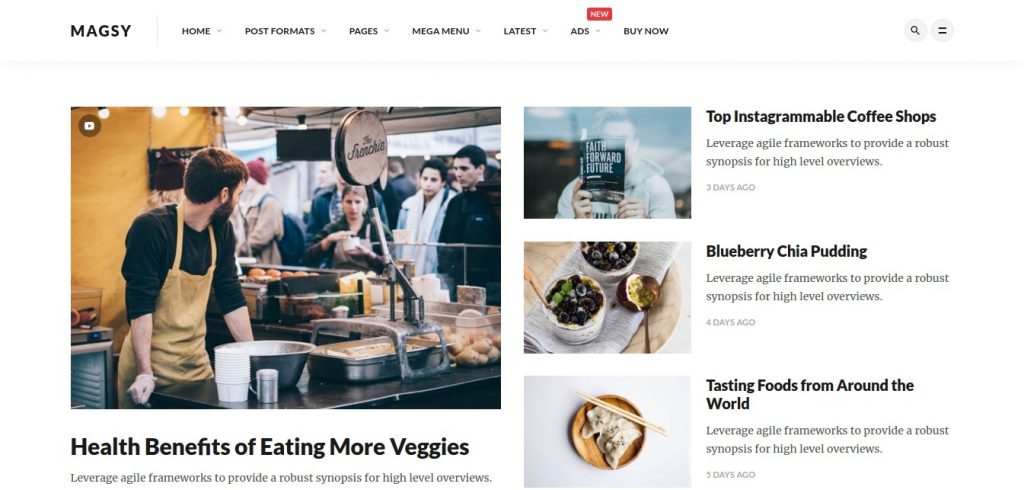*Detailed Caption:*

A screenshot of a webpage is displayed, showcasing the top navigation bar and various sections in detail. In the top-left corner, the page title "Magsy" is highlighted, followed by a series of navigation options. Moving rightward, the menu includes "Home," "Post Formats," "Pages," "Mega Menu," "Latest," and "Ads," each accompanied by a drop-down button. Above the word "Ads" is a conspicuous red rectangular label with "New" written inside it in white text. Further to the right is the option "Buy Now." At the far right of the navigation bar are a magnifying glass icon symbolizing search functionality and a set of two horizontal lines resembling an equal sign.

Beneath the navigation bar, an image captures a lively scene at an outdoor food stand. Behind the counter, a person wearing an apron is engaged with customers standing on the other side. This image is followed by a caption that reads, "Health Benefits of Eating More Veggies." Below this caption, in a smaller font, is the text, "Leverage agile frameworks to provide a robust synopsis for high level overviews."

To the right of this section are three thumbnails, each accompanied by descriptive captions and additional text. The first thumbnail features a man holding up the book titled "Faith Forward Future" with a caption, "Top Instagrammable Coffee Shops," followed by the recurring text, "Leverage agile frameworks to provide a robust synopsis for high level overviews," and a note indicating that the content was posted three days ago.

The second thumbnail displays two jars of blueberry chia pudding set on a napkin atop a wooden serving dish, accompanied by a spoon and what appears to be an open passion fruit with the spoon inserted into it. The caption for this image is "Blueberry Chia Pudding," followed by the same recurring synopsis text, and a timestamp noting it was posted four days ago.

The third and final thumbnail shows a wooden plate with chopsticks laid diagonally across it. Beneath the chopsticks are three steamed wontons. The caption beside this image reads, "Tasting Foods from Around the World," again followed by the recurring synopsis text, and noting that it was posted five days ago.